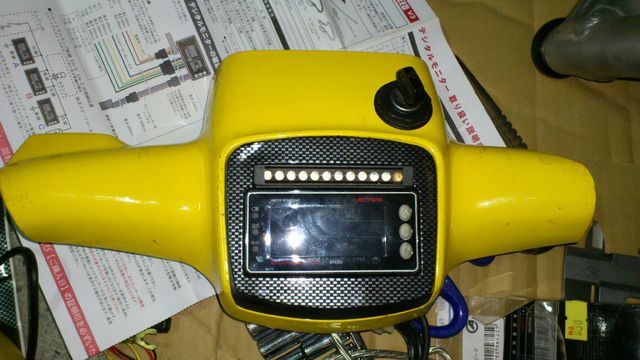The image depicts a black and yellow electronic device, potentially a digital gauge or control module for a motorized apparatus. The black digital face features a display, along with a row of tiny indicator lights positioned at the top. Above the display, there is a small, raised black key-like knob that can be turned left or right. On either side of the device are two dome-shaped mounts, suggesting that it can be affixed to a round object such as an iron pole or handlebars. This entire setup is placed on an instruction manual, which is written in a foreign language and contains red, green, and black text. The manual itself is a white, folded piece of paper. Everything is resting on a piece of brown cardboard, implying that the device is newly unpacked.